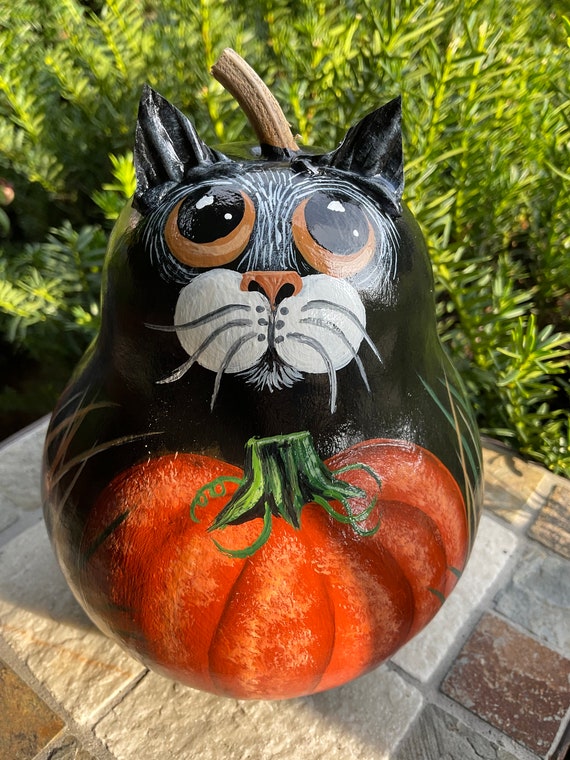This outdoor photo captures a uniquely painted gourd, which resembles a pumpkin, adorned with an intricate black cat design. The pumpkin features a natural woody stem at the top, and black cat ears appear to be taped or glued on. The cat's face is meticulously painted with black fur, contrasting white lips, whiskers, and a few white hairs on its chin and around its face. The cat's light brown eyes add a touch of realism. Below the cat, the gourd is painted orange, mimicking a traditional pumpkin with a green stem, surrounded by painted grass fronds. Set on stone tiles, the scene is enhanced by a backdrop of sunlit, green leafy plants, creating a charming and whimsical outdoor craft display.